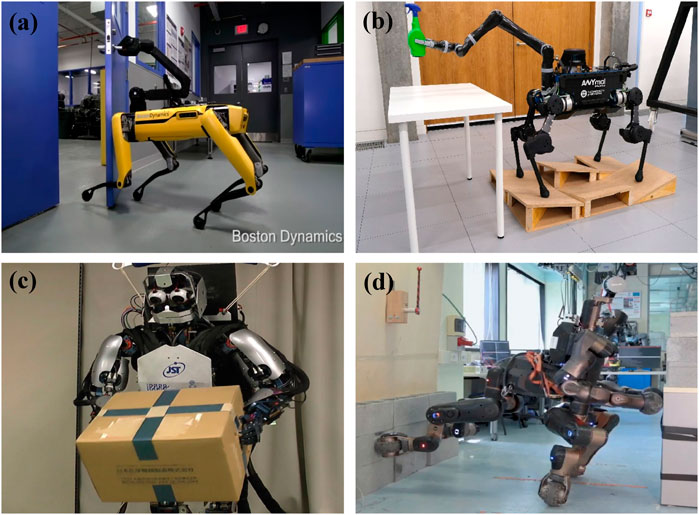The image is a quad compilation of four different robots labeled A, B, C, and D, each situated in their respective quadrants. In the top-left corner (Robot A), a yellow, quadrupedal robot, notably marked with a "Boston Dynamics" watermark, is positioned on a grey floor with blue walls, appearing to open a black door using an arm extending from its top, which gives it a dog-like appearance. To the right (Robot B), a four-legged, black robot is seen standing on wooden pallets near a white table, holding a green cleaning product spray bottle in its gray hand, suggesting a task environment in a white room with brown doors. In the bottom-left quadrant (Robot C), a silver and black humanoid robot with two legs and two arms is holding a brown packing box and has distinctive eye-like features, situated in what seems to be an open space. Finally, in the bottom-right quadrant (Robot D), a robot that is either on all fours or pushing against a wall is seen in an industrial-like area, poised in a manner that suggests it is not engaged in a specific task.